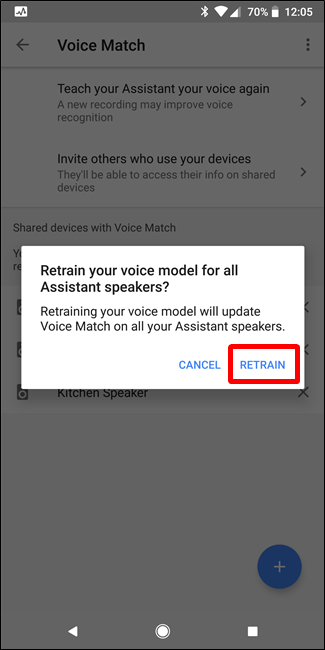The screenshot from the cell phone features several distinct elements. At the top, there is a dark gray border about half an inch thick, transitioning to a light gray due to a pop-up tab overlay, which creates a background effect.

On the top left of the screen, a small white square displays, featuring a black line resembling a heartbeat graph. To the right of this icon, in white text, it reads "1205". Adjacent to this, there is a battery icon indicating 70% charge with the top part in gray and the number 70% written to its left. The status bar further shows three out of four bars full for cellular signal strength, a fully filled Wi-Fi icon, and an active Bluetooth symbol.

Beneath the pop-up tab in the background, the top left corner contains a black left-pointing arrow. Next to it, the text "Voice Match" is visible, with ellipses trailing vertically to the right. A thin line separates this section from the bold black text stating, "Teach your Assistant your voice again." Below are two lines of descriptive information followed by another bold black text, "Invite others who use your devices," with two additional lines of information underneath it. The text "Shared devices with Voice Match" appears next, but further content is obscured by the pop-up tab.

The white rectangle of the pop-up tab itself bears bold black text reading, "Retrain your voice model for all Assistant speakers?" In smaller black text below, it says, "Retraining your voice model will update Voice Match on all your Assistant speakers." At the bottom right corner of this rectangle, there is a red-bordered white circle with a blue "Retrain" button inside, and a "Cancel" button to its left.

A blue circular icon with a white plus sign is located just below the bottom right corner of the rectangle. At the bottom edge of the screen, typical navigation buttons are visible—namely, the back button, the record button, and the start button.